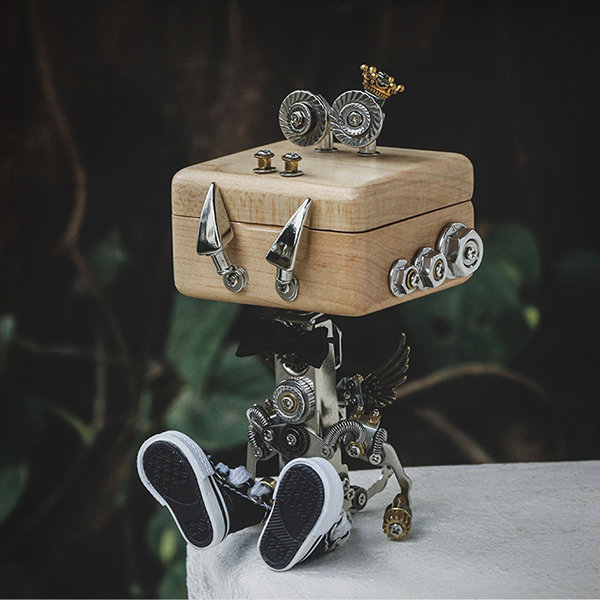In this image, a steampunk-inspired sculpture is prominently displayed on a concrete ledge. The robot-like creation features a square wooden box as its head, crafted from light-colored wood. Various metal elements are integrated into its design: three differently sized nuts and bolts adorn one side of the head, while two small sliver buttons, as well as what appear to be screws, serve as facial features. The body is an assemblage of metal objects, including springs, gears, and even a pair of wings made from dark or pewter-colored metal. A black bow tie adds a whimsical touch. Its feet are fitted with old-style high-top basketball shoes, in classic black and white. Surrounding the sculpture, the background subtly reveals wood twigs, parts of a tree, and some greenery, suggesting a natural, forest-like setting. The range of colors in the image includes green, black, gray, silver, and gold, enhancing the eclectic and artistic nature of the piece. The detailed craftsmanship and blended materials make the robot sculpture the focal point against the contrasting concrete and natural background.